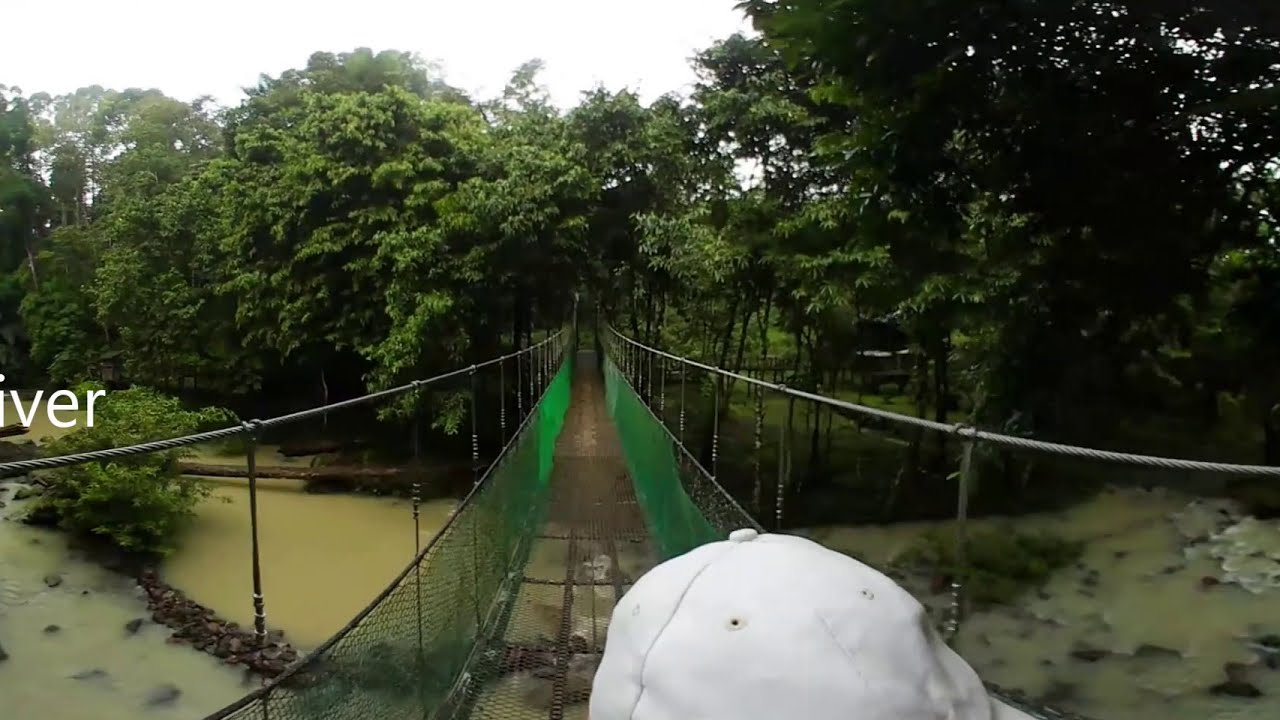In this overcast image, captured possibly with a GoPro, we see the back of a person wearing a white baseball cap as they walk over a suspension bridge. The bridge, characterized by metal wires and posts, features green netting on both sides, functioning as a safety barrier. The flooring appears to be made of mesh, allowing a clear view down to the ground below. Beneath the bridge lies a murky, olive green or brown river, littered with dark gray stones and patches of green shrubbery. Surrounding the scene are dense trees filled with lush green leaves, indicating a warm climate. Natural light filters through the branches and leaves, adding a touch of brightness to the otherwise gray, overcast sky.